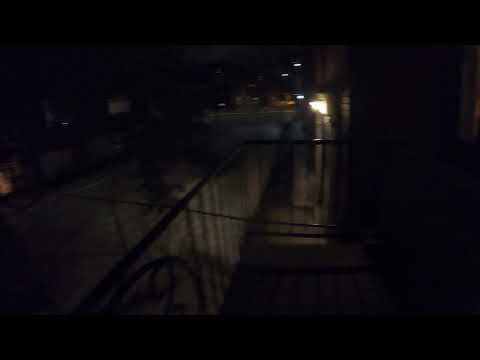The photo is an extremely dark, blurry image, making it difficult to discern details. Approximately 80-90% of the picture is obscured by darkness, contributing to the challenge of identifying specific elements. Though poorly lit, the scene appears to be an external urban setting, possibly taken at night. There is a suggestion of a balcony or porch overlooking what might be an entrance way, marked by a faint light source that casts minimal illumination. 

In the bottom left corner, a black-colored fence of the balcony and potentially a chair are faintly visible. A pathway appears to lead from the vantage point towards a doorway, illuminated by another dim light. Beyond this pathway, there is an indication of a road and some buildings, including a light brown one and a dark gray one. A gate is also mentioned, which may serve to prevent entry. Despite the clues, the exact details remain ambiguous due to the overarching darkness and lack of focus in the image, leaving the impression of an urban, perhaps industrial, setting shrouded in night fog.